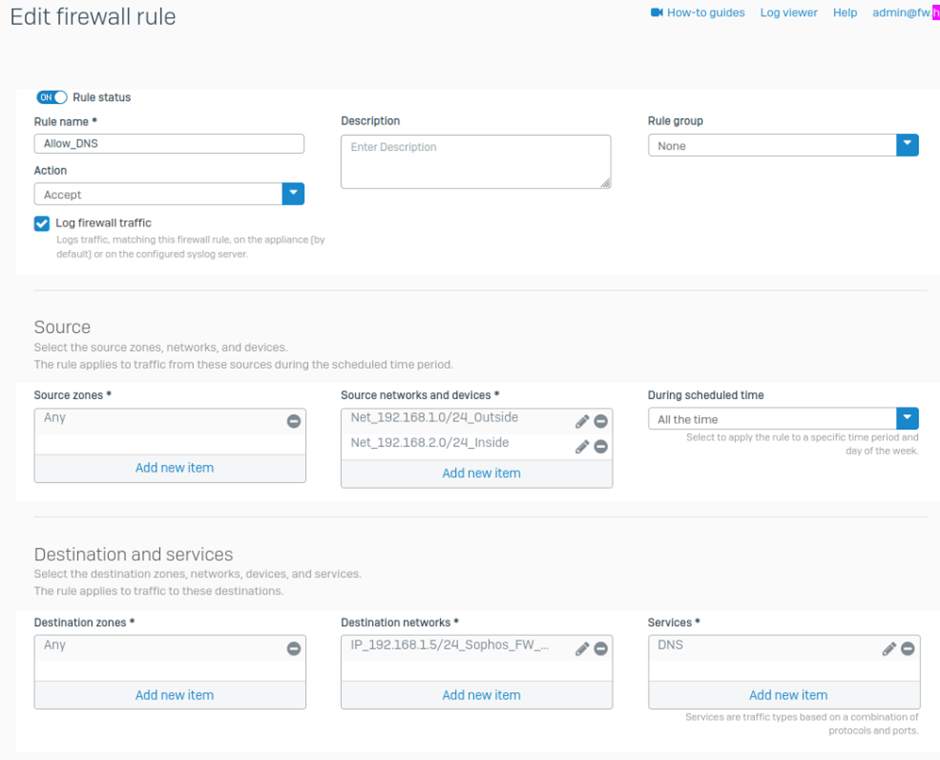The image displays a dialog screen titled "Edit Firewall Rule." This screen is designed for modifying or creating firewall rules for a device, such as a personal laptop or computer, or potentially for an entire network. Directly to the right of the title, a series of tabs are visible, including "How-To Guides," "Log Viewer," "Help," and a tab that provides an email link to the site admin. Below these tabs, there is a list of various rules that can be toggled on or off. The interface is divided into sections: one labeled "Source," where users can select source zones, networks, and devices, and another labeled "Destination and Services."